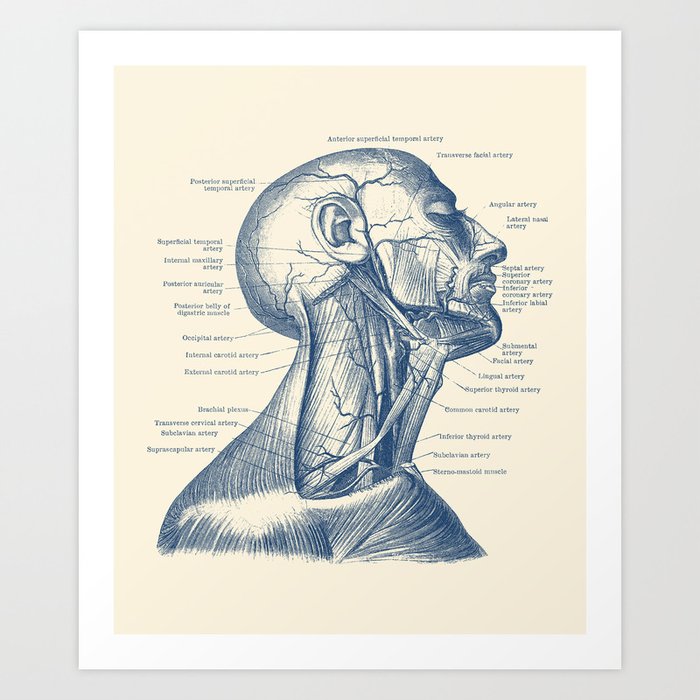The image is a detailed anatomical print, likely intended for educational purposes such as medical studies. It features a blue or dark blue depiction of the human upper body, specifically from the top of the skull down to slightly below the shoulders, all set against a flesh-colored or light pink background. The subject is a side profile of a male figure with his head slightly tilted, revealing an intricate view of the venous and circulatory systems along with muscles and tendons. Multiple lines connect various labeled points to specific parts of the anatomy, including arteries like the occipital artery, internal carotid artery, external carotid artery, angular artery, and transverse facial artery. There are approximately 20 different body parts noted. The image is framed with thick gray and white borders, making the inner details stand out. The precise labeling and detailed depiction suggest that this image is used for medical learning and examination preparation.